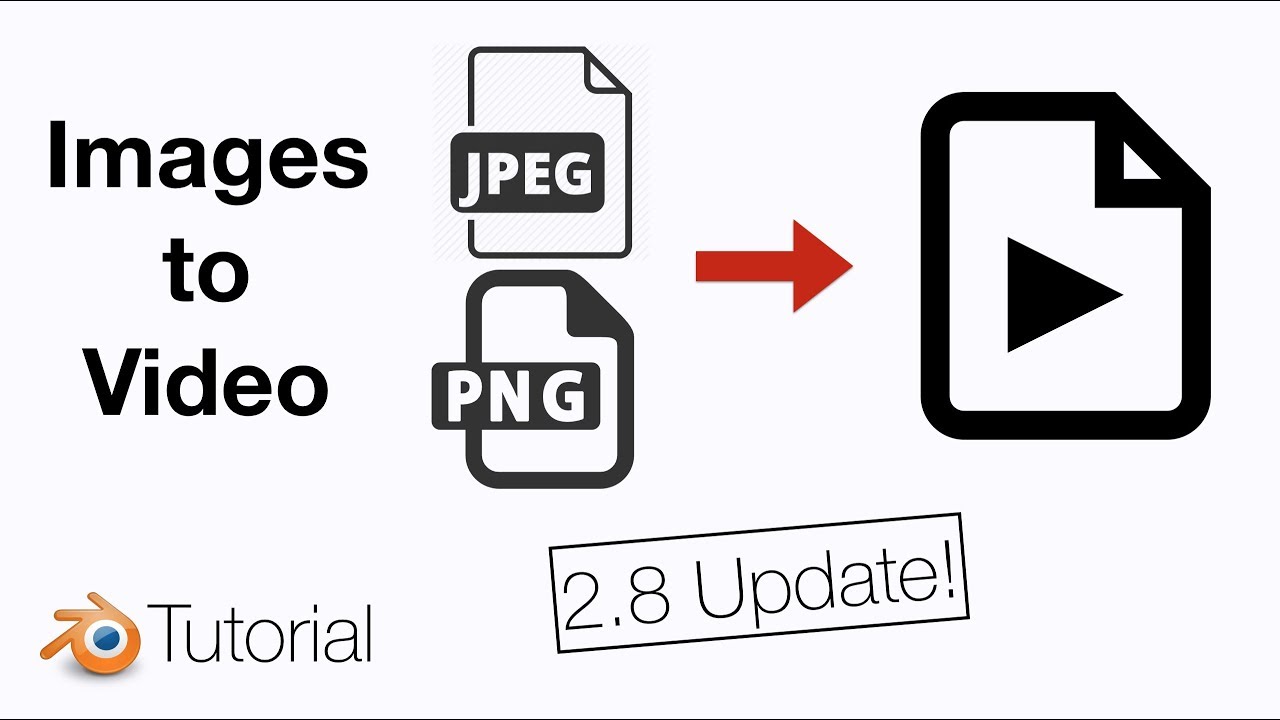The image is a detailed digital thumbnail with a whitish-gray background. There are black lines at the top and bottom edges, and the content is organized horizontally. 

On the left side, the black text reads "images to video." Below this, there are two icons resembling pieces of paper with their top right corners folded. The top icon has "JPEG" written in white text, and the bottom one has "PNG" written in white text. 

To the right of these icons, a red arrow points to the right. Following the arrow, there is another piece of paper icon with a folded corner displaying a black, sideways triangle in the center, representing a play button.

Below this central arrangement is a black-outlined rectangular box that reads "2.8 update!" in black text. Additionally, in the bottom left corner, there is a blue circle with what appears to be eyelashes, surrounded by a white border and set against an orange background. This emblem accompanies the word "tutorial."